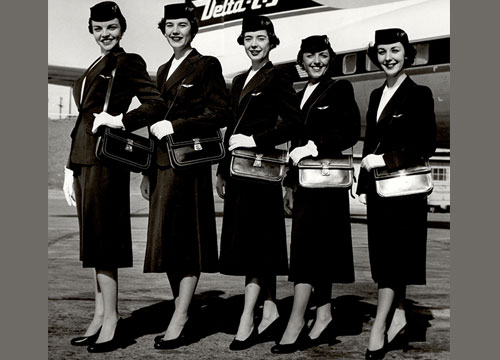This vintage black-and-white photograph features a line of five women who are flight attendants, historically referred to as stewardesses, standing in front of a Delta aircraft. Each woman is clad in a coordinated dark uniform consisting of a knee-length skirt, a tailored coat, and a white shirt underneath. They each wear a pair of black pumps and a dark-colored cap atop their short, dark hair. 

Notably, on the left lapel of their coats, you can discern the light-colored shape of wings badges, indicating their role. Their dark leather purses, complete with a central buckle, are slung over their left shoulders, with their left hands resting on top of the purses. Each flight attendant stands with her left side closer to the camera, left foot slightly forward, but they have turned their heads to gaze directly at the lens.

In the background, a section of the airplane's rear is visible. The aircraft’s tail fin prominently displays the word "Delta" in white letters. The plane itself shows distinct color segmentation, with a white top, a black area around the windows, and a darker lower section. The sky forms a subtle backdrop to this organized and poised group.